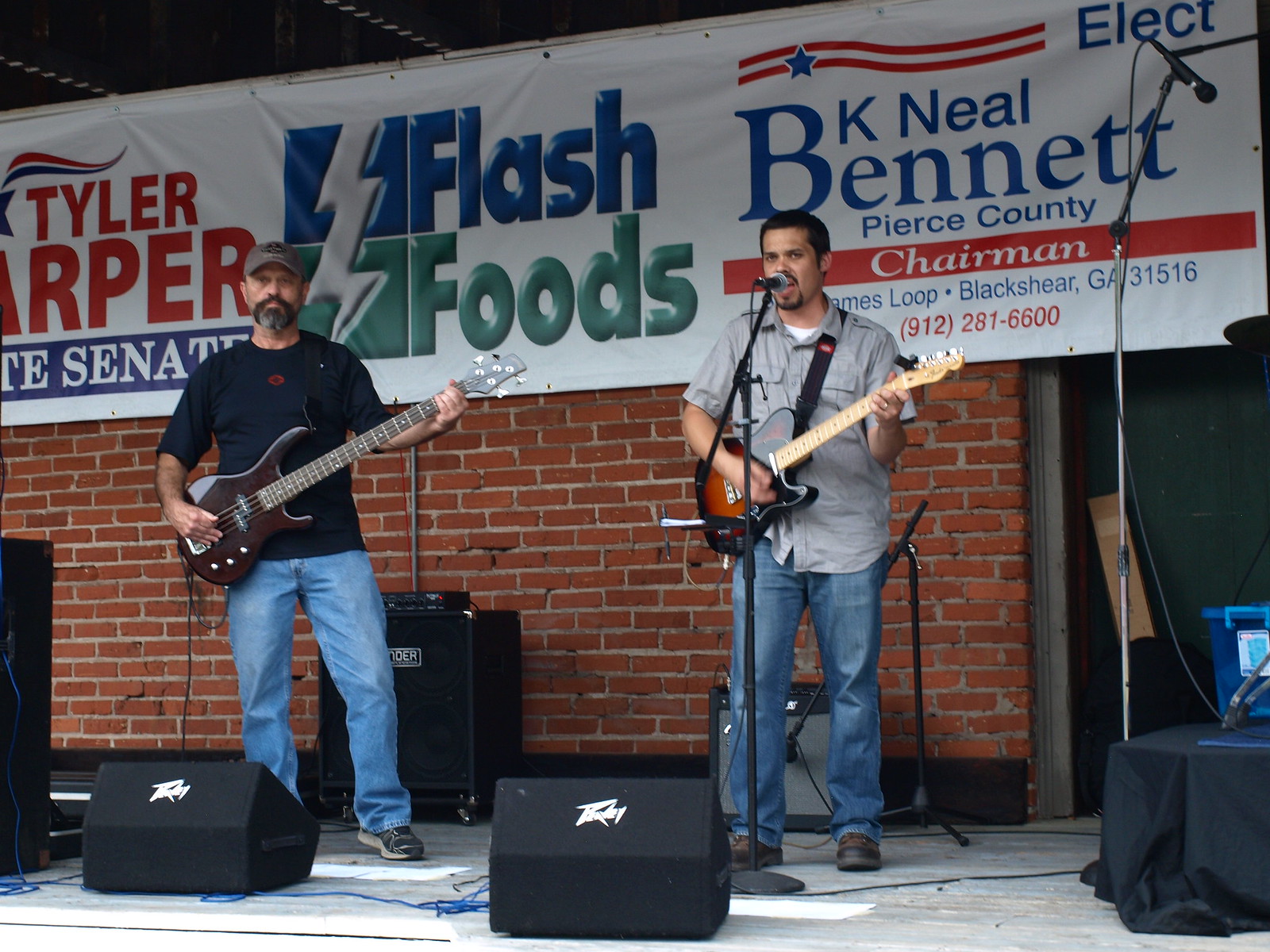The image portrays a lively musical performance captured from the audience's perspective, seemingly right in front of the stage as no spectators are visible in the foreground. The setting features two musicians prominently positioned. The man on the left, an older white man with a beard and a hat, is dressed in a navy short-sleeved t-shirt rolled up at the elbows, blue jeans, and sneakers, handling a brown or deep maroon bass guitar. On the right stands a Hispanic man with dark hair and a black goatee, sporting a gray button-down shirt, blue jeans, and work boots. He is playing a Telecaster guitar and singing into a microphone.

The stage setup includes Peavey speakers positioned at the front, accompanied by a backdrop of red brickwork with a large white banner advertising local businesses. The banner prominently displays a logo for "Flash Foods" featuring a lightning bolt and electoral promotions that read "Re-elect B.K. Neil Bennett, Pierce County Chairman" and part of a Senate advertisement. Amplifiers of varying sizes are visible behind the musicians, adding to the authentic concert atmosphere.